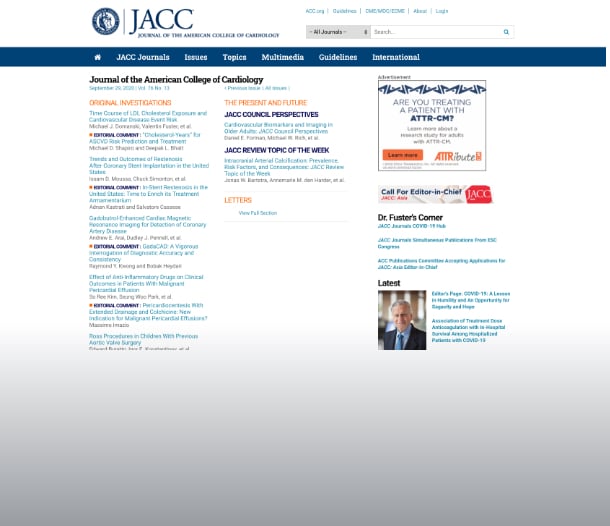In this screenshot of the JACC website, the layout is meticulously organized, starting from the top. To the right side, five small categories are displayed in a distinct blue color. Below these categories is a prominent gray rectangle, adjacent to which lies a search bar for easy navigation. Following these elements, the website’s primary categories are listed in white text: JACC Journals, Issues, Topics, Multimedia, Guidelines, and International.

Heading the main section is the title "Journal of the American College of Cardiology." On the left side, a list of blue links under the heading "Original Investigations" in orange is visible. Featured prominently to the right is the section titled "The Present and Future" in orange, with two articles listed beneath it.

Below this, there's a smaller section titled "Letters," containing a solitary clickable blue link. The site’s background transitions smoothly from gray at the top to white further down, creating a clean and professional visual appeal. 

On the right side of the webpage, an advertisement asks, "Are you treating a patient with ATTRCM?" with a call-to-action button that says "Learn More" in an orange rectangle. Beneath this ad, there is a "Call for Editor in Chief" announcement. Further down, a section titled "Doctor's Corner" features three click-worthy blue links. Another segment, labeled "Latest," includes an image that appears to be of a politician or doctor, accompanied by two related blue links to the right of the image. This completes the comprehensive overview of the image captured from the JACC website.